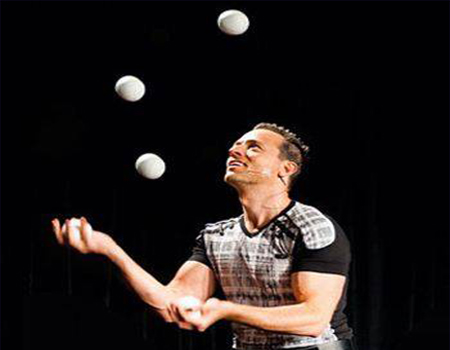In this striking image, a muscular, clean-shaven Caucasian man with shortly cropped black hair stands on a stage, illuminated against a completely black background. He is juggling five white balls, each roughly the size of tennis balls. Three balls are suspended mid-air, with one ball held in each of his hands. His head is tilted back, eyes focused upwards with a broad smile, conveying his enjoyment and engagement with the performance. The man is wearing a tight-fitting black shirt adorned with a distinctive black and white checker-like pattern on the front. The shirt accentuates his well-defined biceps. A small, thin microphone attached to his ear indicates that he is in the midst of an on-stage show, allowing him to move fluidly and speak to the audience simultaneously. The lighting is sharply concentrated on him, highlighting his presence and making him the central focus of the scene.